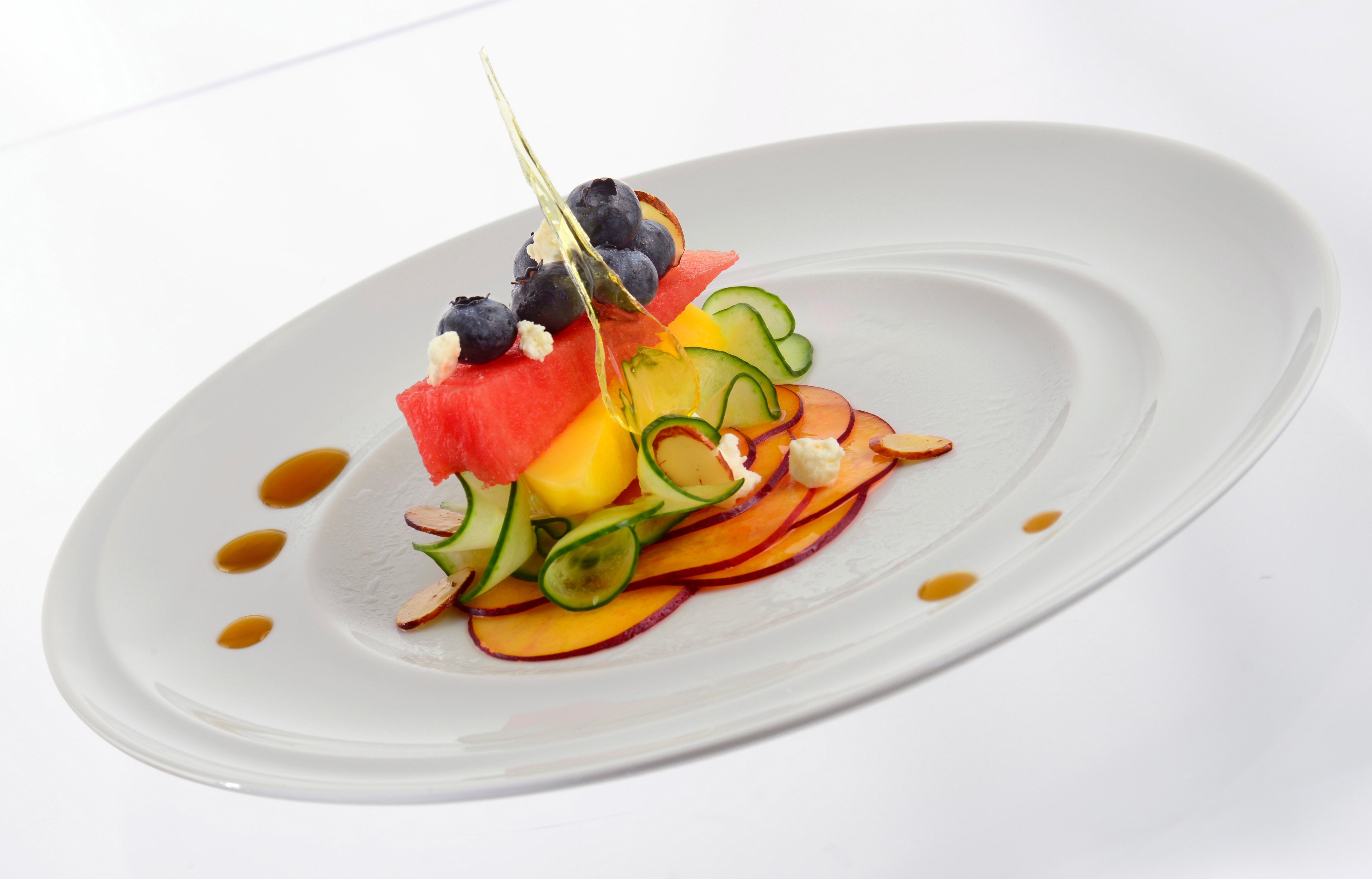On a plain white plate, there is an elegantly arranged appetizer composed entirely of sliced fruits and vegetables. The base consists of thinly sliced peach or yellow squash with a red border, topped with neatly arranged circular slices of lime. Above this layer, there are pieces of orange melon and watermelon stacked, crowned with several fresh blueberries. The dish is adorned with an artistic touch: five strategic drops of a brown sauce, possibly honey, placed along the edges of the plate, enhancing its gourmet presentation. To add to the visual appeal, a ribbon-like curl of green cucumber is elegantly incorporated into the arrangement.